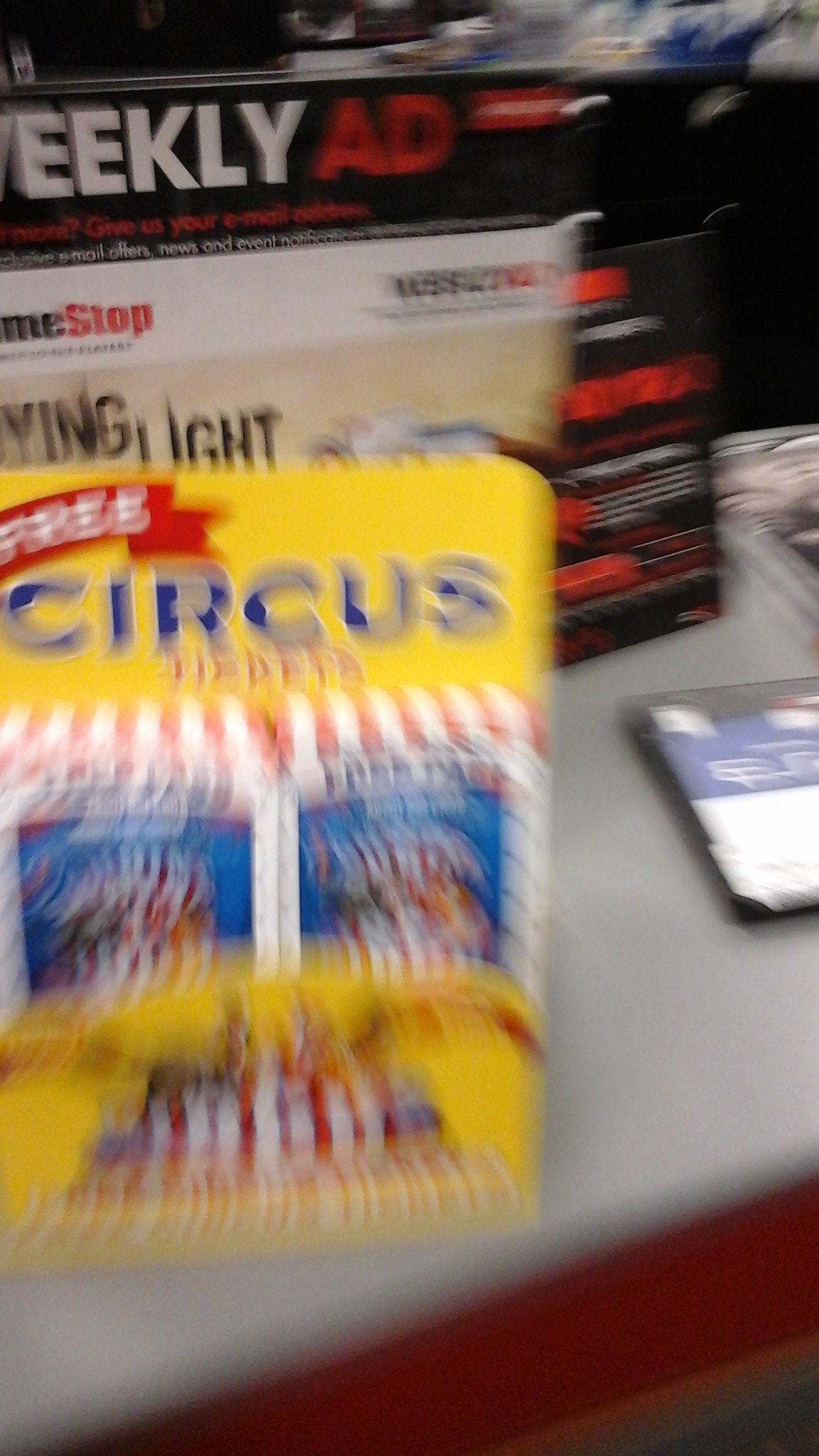The image is a vertically oriented photograph that is significantly blurred. In the background, there is a box labeled "Weekly Ad" with black, white, and red lettering. In the foreground, the narrow countertop, likely made of a plastic material, appears white. A black smartphone displaying a blue and white screen rests on the right-center area of the countertop.

Dominating the left-center to the middle of the image is a package or box titled "Free Circus Tidbits." This object features three photographs depicting circus scenes, characterized by prominent red and white striped elements. The background color of this package is yellow.

Leaning against this package is another box, positioned upright, with a black and white design. It features text in red, black, and white. This second box is labeled "Game Stop" and includes the phrase "Flying Light." 

Despite the overall blur, the composition and items suggest a setting filled with promotional packages and modern electronics.